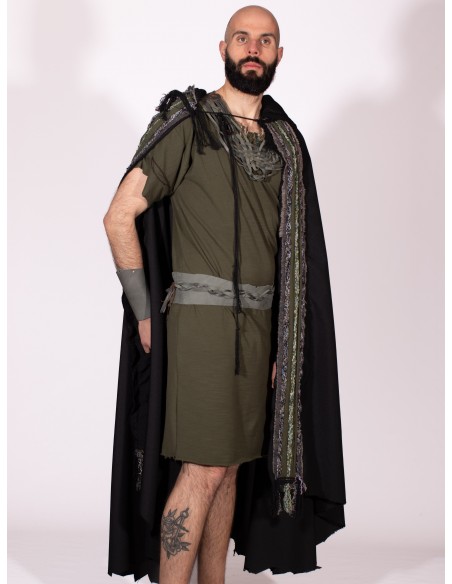The photograph features a white or Caucasian man with light skin, a bald head, and a dark brown mustache and beard. He has a serious, almost menacing facial expression and stares straight ahead into the camera. He is dressed in a green robe that extends to his knees, resembling medieval or Roman-style festival attire. The robe is secured with a gray belt around his waist, and it appears slightly frayed at the top. Draped over his left shoulder is a dark green cape with ridged fabric on the sides, fastened with a string around his left shoulder. He also wears gray bracers on his wrists. Notably, he has a large tattoo on his right leg, depicting an anchor with a dragon wrapped around it. The photo is taken in front of a white backdrop, with gray shadows visible in the top right corner and bottom, emphasizing the indoor setting.